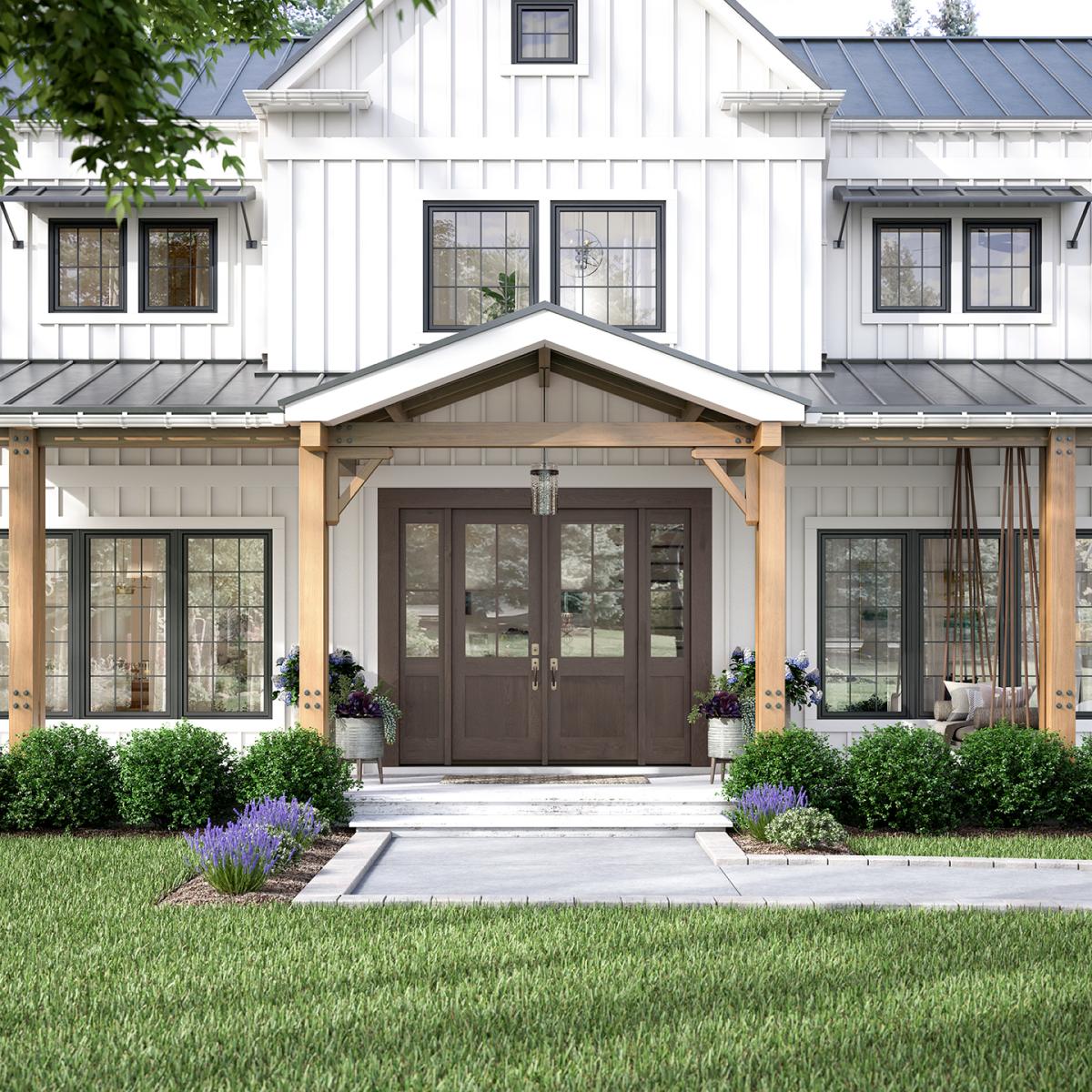This image showcases the exterior front of a picturesque, two-story, white American suburban home with a well-manicured, vibrant green lawn. The lawn surrounds a concrete walkway that leads directly to the front entrance, which comprises elegant white steps ascending to a cozy front porch. The porch, characterized by its gray tiling and a V-shaped roof, features a symmetric design with a rustic porch swing on the right side and a centrally hanging light fixture illuminating the space. The house’s double-entry front doors are a rich brown, accented by small side windows on either side, adding to the aesthetic symmetry.

Potted flowers grace both sides of the archway leading to the doors, contributing to the home's welcoming ambiance. Along the walkway, neatly trimmed round bushes and vibrant flowers, set in mulched beds, enhance the garden's charm. The upper level of the house features six windows – two on the right, two in the middle, and two on the left – with a small attic window perched at the top. The windows are contrasted with black framing, and are mirrored below by additional ground-floor windows.

The roof, a mix of gray and light blue tones, complements the house’s classic white exterior. This harmonious blend of colors and symmetric layout, along with the well-kept garden, project a serene and inviting atmosphere, typical of an idyllic suburban setting.